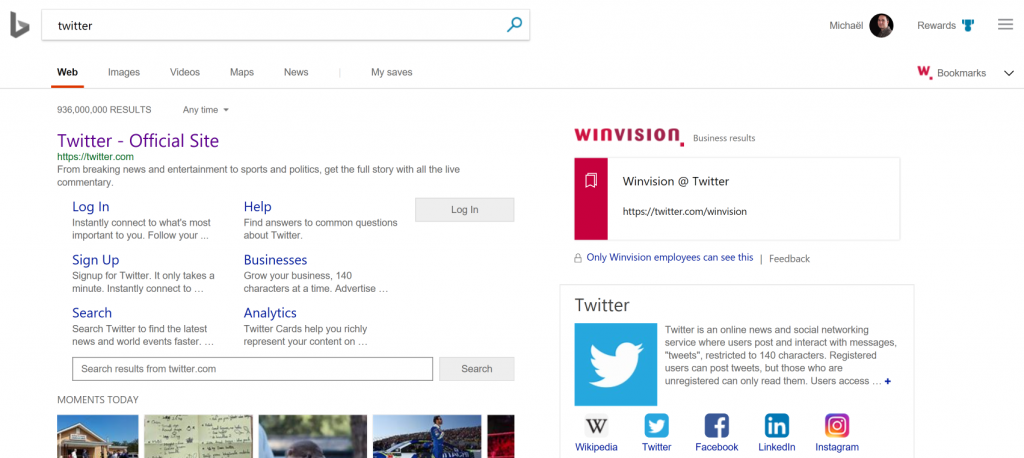The image displays a Bing search results page featuring the Twitter website. On the far left-hand side, the Bing logo is prominently visible, resembling an overturned 'V' with a line creating a stylized 'B', conveying a futuristic aesthetic. 

In the top-right corner, there is a small black circular icon displaying a light-skinned person wearing a gray shirt, indicating the user, named "Míchael", with an accent over the 'E'. Next to the user's name, the navigation bar displays the word "Rewards" in black text, followed by a blue award icon with a ribbon. Below this, there is a "Bookmarks" section marked with a red 'W' and a dot, written in black text, accompanied by a black arrow pointing to the right.

On the left-hand side of the page, a white search bar with a cyan blue magnifying glass icon on the right is visible. The search bar currently contains the term "Twitter," spelled out as T-W-I-T-T-E-R. Above the search bar is a navigation menu, segmented into six tabs: 'All,' 'Images,' 'Videos,' 'Maps,' 'News,' and 'My Saves,' with the 'All' tab currently selected.

The search results highlight the official Twitter website. Under a header that reads "Twitter - Official Site," the URL is displayed in hyperlinked blue text. Beneath this, additional links include "Login," "Help," "Sign Up," "Business," "Search," and "Analytics," all presented in the same blue hypertext. The image also includes a small icon of a house and a few other elements at the bottom, completing the detailed depiction of the Bing search results interface.